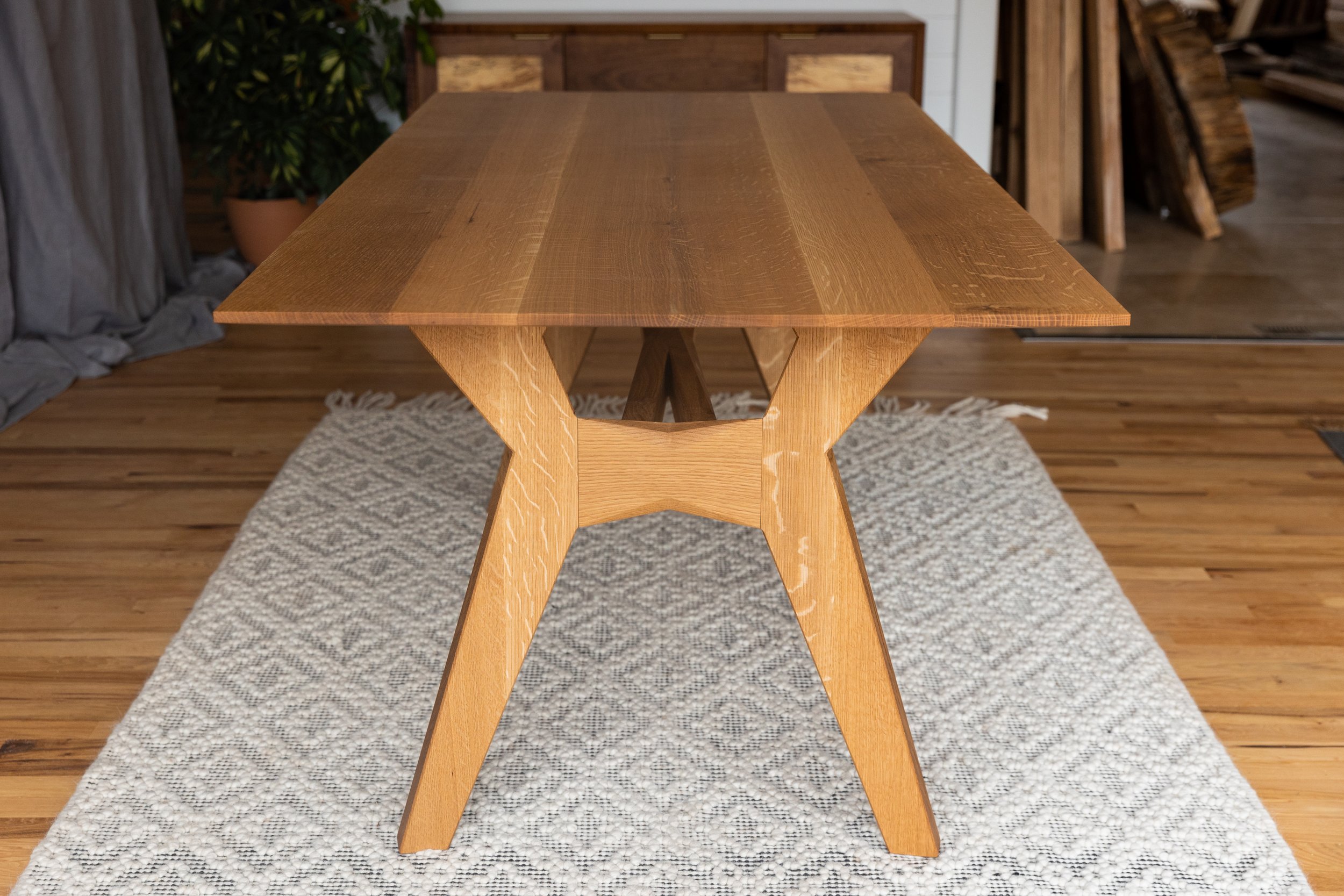In this detailed image, a light wooden table sits centrally on a gray rug featuring a diagonal, diamond-shaped pattern. The gray rug contrasts with the underlying clean, wooden floor tiles that run horizontally. The table, made from six thick wooden panels, is long enough to comfortably seat four people. Despite some scratches on its surface, the table maintains a polished appearance. In the background, a dresser displays additional wooden objects and long wooden planks, hinting at a workshop or showroom setting. Adding a touch of nature, a plant in a wooden pot is placed alongside the dresser, blending harmoniously with the wooden elements in the scene.